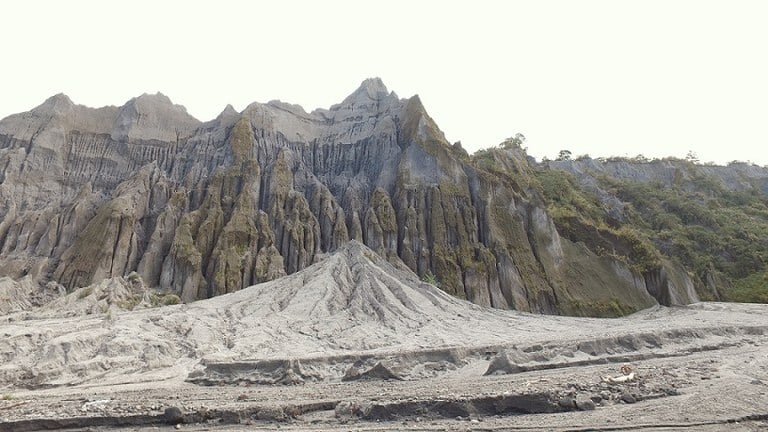This photograph captures a captivating mountainous landscape under a cloudy, whitewashed sky. In the foreground, there is a mound with a texture akin to grain, appearing either as salt or sand with a whitish hue. Further down are scattered rocks, pebbles, and grains, hinting at a gravelly surface, possibly part of a long gravel road, suggesting some machinery might have traversed the area. The middle ground features a shorter, pointy mountainous formation, characterized by its jagged, triangular peaks. On the right, lush patches of grass and trees are dispersed along the mountainside, adding a touch of greenery to the scene. The background reveals taller, rocky mountains in shades of brown and gray, standing 20 to 50 feet away, their pointed tops piercing the dull, muted sky.